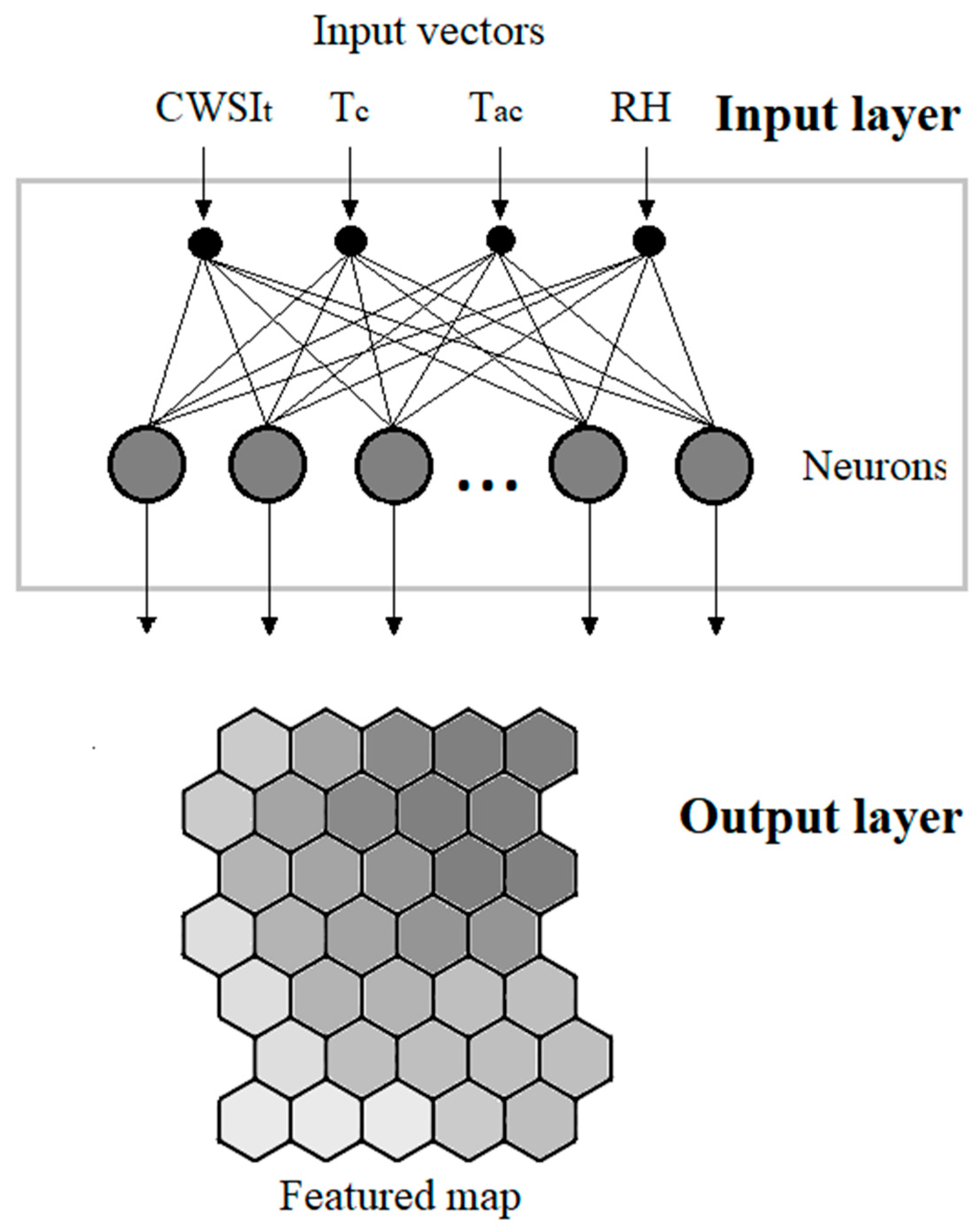The image depicts an illustration commonly found in educational materials, likely related to neural networks or machine learning. At the top of the grayscale image, the text reads "Input Vectors," followed by a rectangular area with four black circles, each associated with specific letters: "CWSI (small t)," "T (small c)," "TAC," and "RH." Each letter arrangement indicates an input vector, which is part of the "Input Layer."

Arrows extend from each of these four black circles, leading downward to connect with five larger gray circles, labeled as "neurons." These gray circles are situated within the outlined rectangle. Further arrows extend from the neurons, pointing outside the rectangle towards a section labeled "Output Layer." Beneath the "Output Layer" label, the term "Featured Map" is prominently displayed, accompanied by a honeycomb-like infographic. This hexagonal pattern starts with lighter gray shades at the bottom left corner, progressively darkening towards the top right corner.

Overall, the detailed diagram emphasizes the flow of data from input vectors through neurons and finally to the featured map in the output layer, visually highlighting the process in a neural network system.